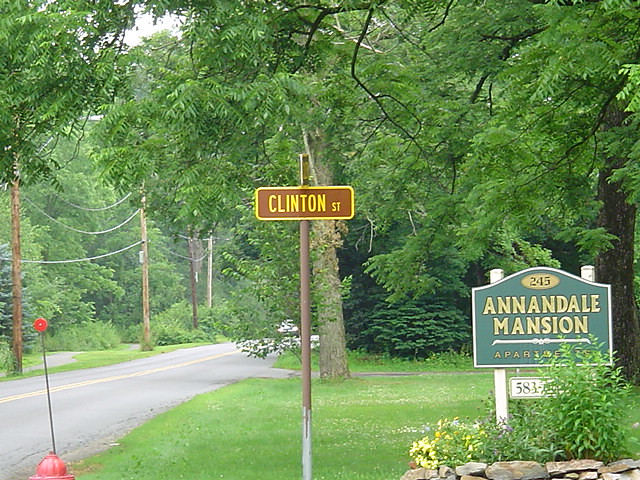In the center of the outdoor image, a rectangular street sign prominently stands on a pole. The pole is uniquely colored, with the top half being brown and the bottom half gray. The sign itself has a distinct yellow border with a brown background and features the text "Clinton, ST" spelled out in yellow. In the backdrop, a lush, green field of grass stretches out, adding a vibrant touch to the scene. The bottom right corner of the image is adorned with a variety of plants and flowers, accompanied by some scattered rocks. In the distant background, partially visible, is another sign, which reads "Annadel" spelled A-N-N-A-D.